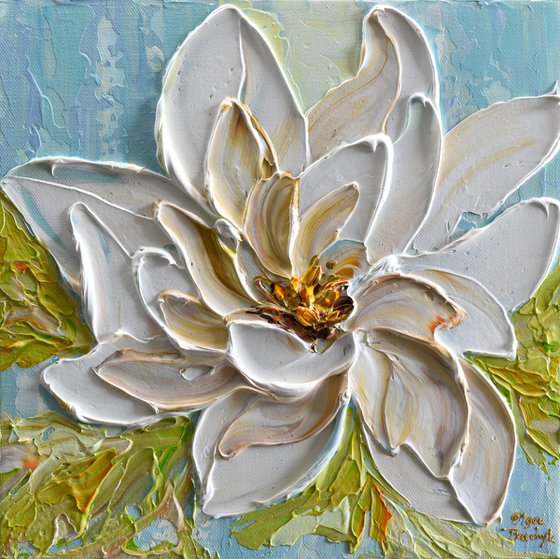The image portrays a close-up of a textured artwork, likely an oil painting or a relief, featuring a large, white magnolia flower as the central focus. The petals of the magnolia are adorned with slight yellow or gold streaks, transitioning to a center that exhibits hues of yellow and brown. The flower is surrounded by green leaves set against a dynamic background that combines shades of blue and white, evoking a sky-like effect, with touches of green suggesting grass below. The background appears rough and textured, adding to the overall depth and tactile quality of the piece. Small tinges of light orange and a hint of pink can also be observed in the composition. The artist's signature in the lower right corner is written in a light golden or green color, but the name remains indecipherable, with identifiable letters being "G-R-E" in the first name and a last name ending with "K". There is no other text or numbering on the artwork.